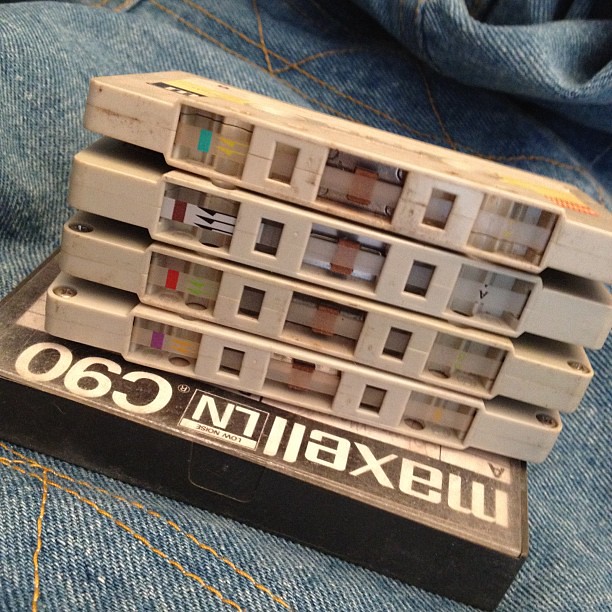In the center of a square color photograph, several beige plastic cassette tapes are meticulously stacked, with their top edges—showing the exposed tape film—facing toward the viewer. These analog tapes are resting on a Maxell cassette case, identifiable by its upside-down text: "Maxell" and "L-N" within a white bordered rectangle, signifying "Low Noise." The case, which prominently displays "C90" among other details, sits on a backdrop of light blue denim fabric. The denim, featuring traditional goldish-brown stitching, adds a textured and nostalgic feel, accentuated by the pocket's triangular stitching patterns visible in the bottom left and upper right corners. From top to bottom, the tapes display a variety of pre-tape identifiers: a blue bar, a white bar with black arrows, a clear bar with green arrows, and a final bar that appears yellow with purple arrows, each housed in its respective brown felt center. The scene encapsulates a tactile sense of vintage media against the rugged, everyday material of denim.